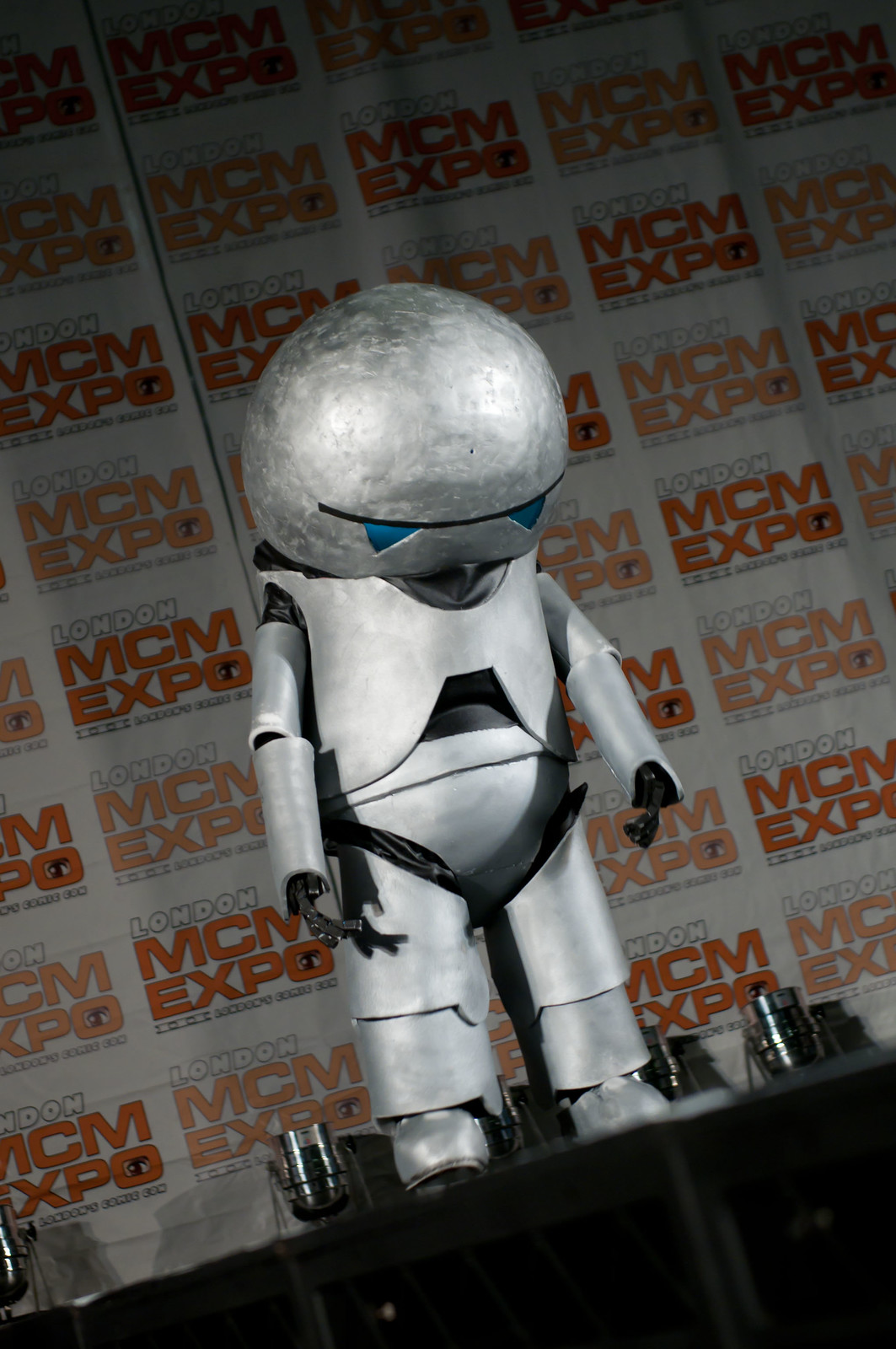This color photograph captures a close-up of a two to three-foot tall, silver robot that seems to straddle the line between art and cosplay. The robot stands diagonally framed at the center of the image on a black stage or table. It possesses a large, round head devoid of facial features save for a thin black line and two blue fang-like triangles, potentially representing eyes, giving it a somewhat "depressed" look as it gazes downward. This "Paranoid Android"-inspired figure appears to have a segmented design: plates cover its chest, lower torso, arms, and legs, along with small black claws for hands and silver shoes. The entire costume, appearing spray-painted, suggests a homemade quality. At its feet, small, smoke-colored glasses rest on the table. The backdrop behind the robot is emblazoned repetitively with "London MCM Expo" in shades of orange and light orange, indicating it might be part of a cosplay convention or promotional event.